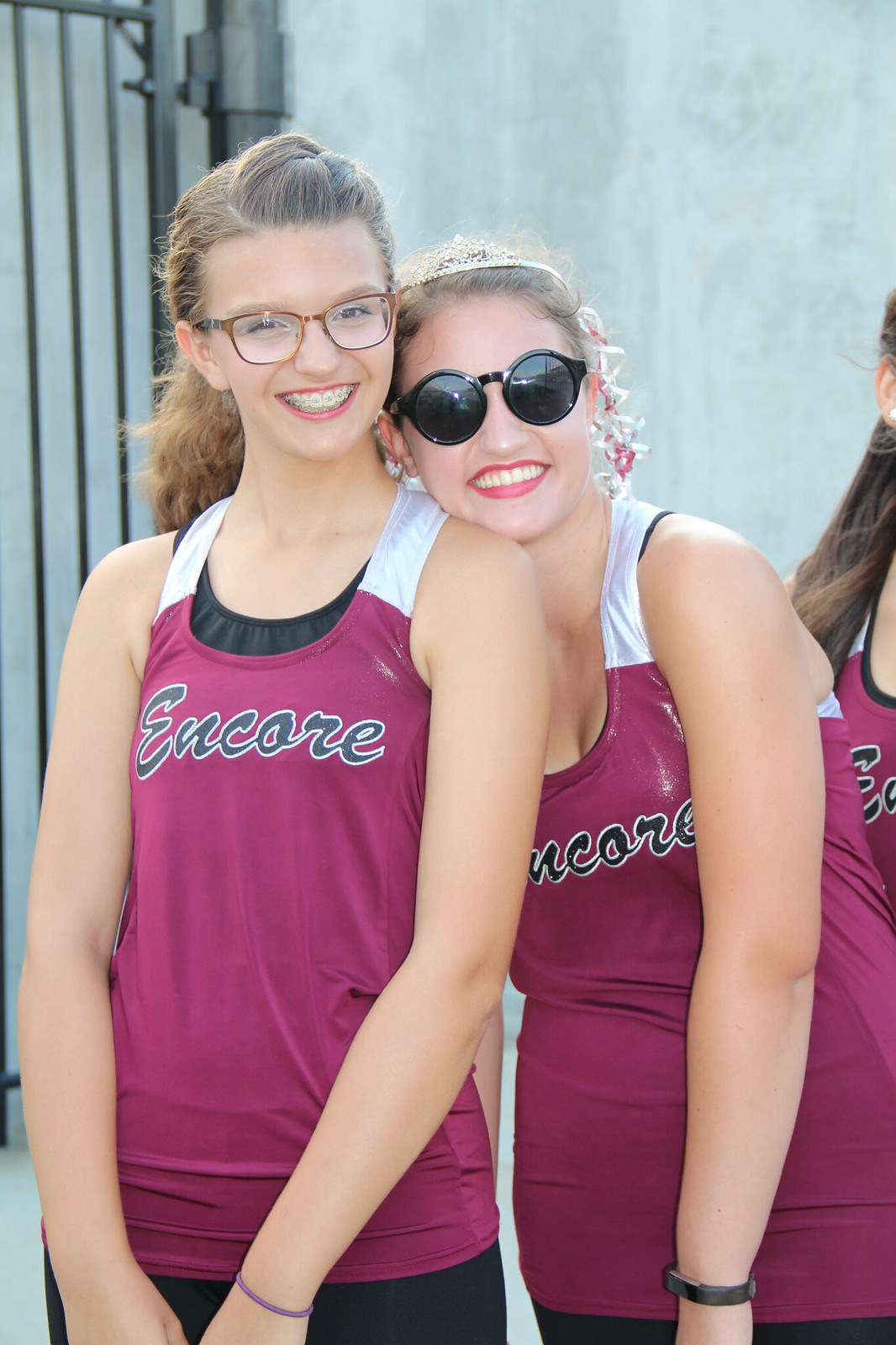In a vibrant scene, two young women are prominently featured wearing sleeveless tank tops with wide white shoulder straps and glittery, reddish-pink fabric emblazoned with the word "Encore." The woman on the left, sporting brown hair in a ponytail, grins brightly, revealing her braces and gold-brown framed glasses. Beside her, the woman on the right, with similarly brown hair, wears dark round sunglasses that obscure her eyes, a small crown, and curly ribbons in her hair. Both have bracelets, with one possibly wearing a watch. Their cheerful expressions radiate joy as they pose closely together, with the woman in sunglasses resting her head on the other's shoulder. Partially visible in the frame, another figure can be seen slightly out of focus, revealing only hair and an earring. The scene is set against a backdrop of a cement sphere and a metal gate, suggesting an outdoor location.